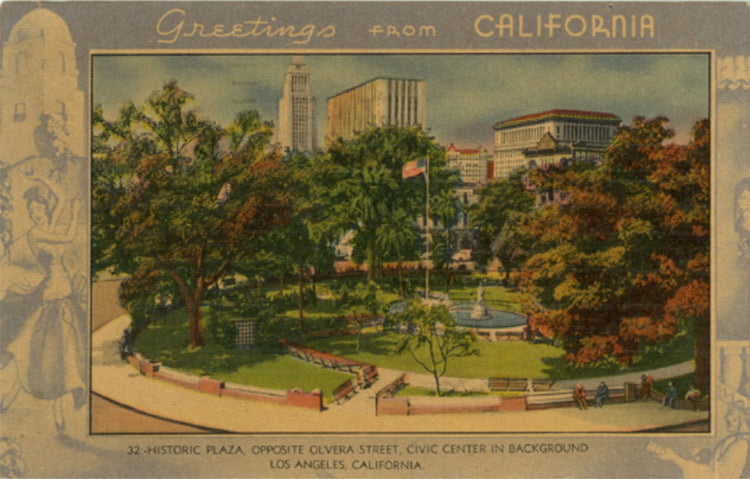This postcard from California, labeled "Greetings from California" in a light brown serif text, appears quite old and carries a sepia-toned appearance. The centerpiece of the postcard is a historic image of 32 Historic Plaza opposite Olvera Street with the Civic Center in the background, Los Angeles, California. The scene depicts a circular park graced with abundant trees, including redwoods, and a prominently featured fountain at its center. An American flag waves proudly either from within or just behind the fountain. The park is bordered by walkways and a large surrounding path or street, with visible figures providing life to the image: a woman in a revealing dress dancing on the left and an elderly man in a sombrero playing guitar on the lower right. The upper background showcases a mix of tall office buildings and skyscrapers, adding depth and context to this vintage Californian setting.